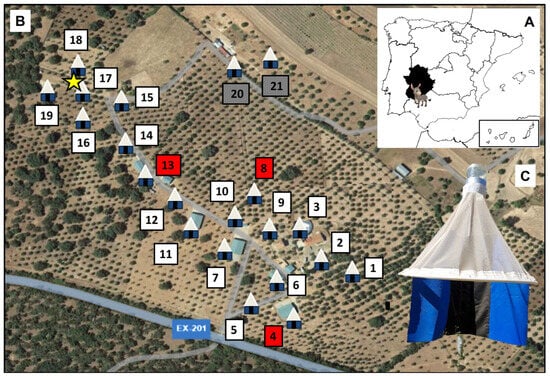This top-down aerial photograph, seemingly taken from a satellite or a platform like Google Earth, showcases a predominantly brown terrain interspersed with green patches of trees. The image is marked with various geometric figures and annotations. Several white squares, some numbered sequentially from 1 to at least 21, are placed across the landscape. Among these are also red and gray squares. On closer inspection, a star is noticeable within one of the squares.

Roads cut through the area, with one diagonal road in the bottom left, another through the middle, and another in the upper right section. Tiny blue structures with triangular white roofs, resembling huts or tents, are scattered across the ground and also labeled within the squares. 

In the top right corner, a white map with black lines outlines a satellite view of a region, marked with a bold "A" and a darkened area. An animal image is present near this map. Directly below, in the bottom right corner, an edited image of a blue and cream tent with a tall triangular roof is depicted. This detailed layout provides a comprehensive view of the terrain with its annotations and structures.